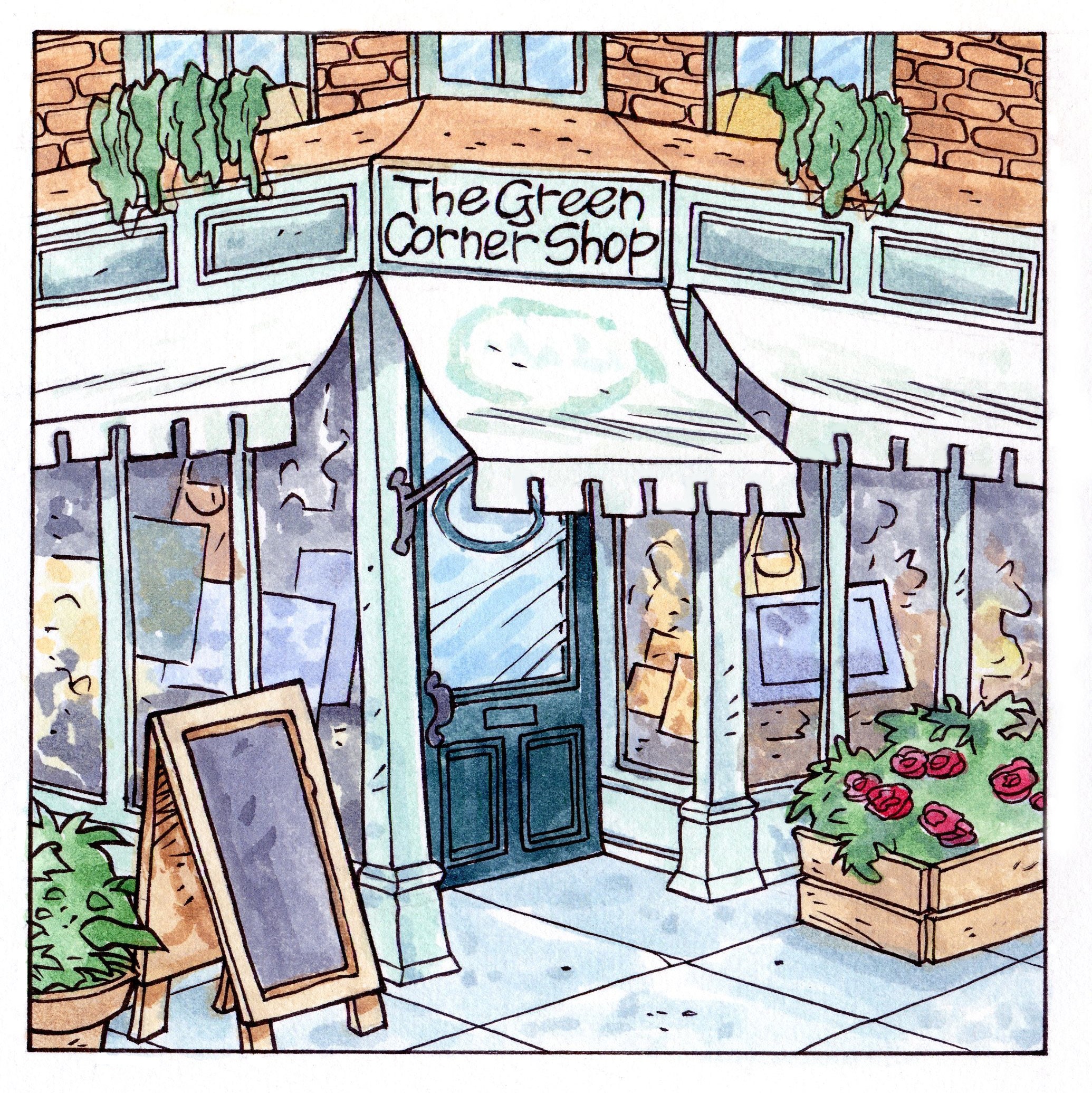This image, a detailed illustration reminiscent of a watercolor painting, depicts a quaint corner shop in an urban setting. The shop, named "The Green Corner Shop," is housed in a charming brick building with an apartment above and a storefront below. The storefront features full glass windows and white canvas awnings extending over both the door and windows on either side of the corner. The shop's dark marine blue door, positioned at the corner, is adorned with a circular glass pane.

Prominently displayed above the awning is the shop's name, "The Green Corner Shop," inscribed in dark letters against a light gray or green background. The window displays suggest it is a gift shop, showcasing purses, posters, and various art pieces. In front of the shop, there is a wooden planter box filled with red flowers, likely roses, positioned near the right-side window. Additionally, a large potted green shrub stands near the left corner of the entrance.

A chalkboard sign, devoid of any writing, stands on the sidewalk, possibly indicating that the shop is closed. Above the shop, the second story features three windows, each adorned with planter boxes spilling green plants over the edges, enhancing the building's inviting charm.